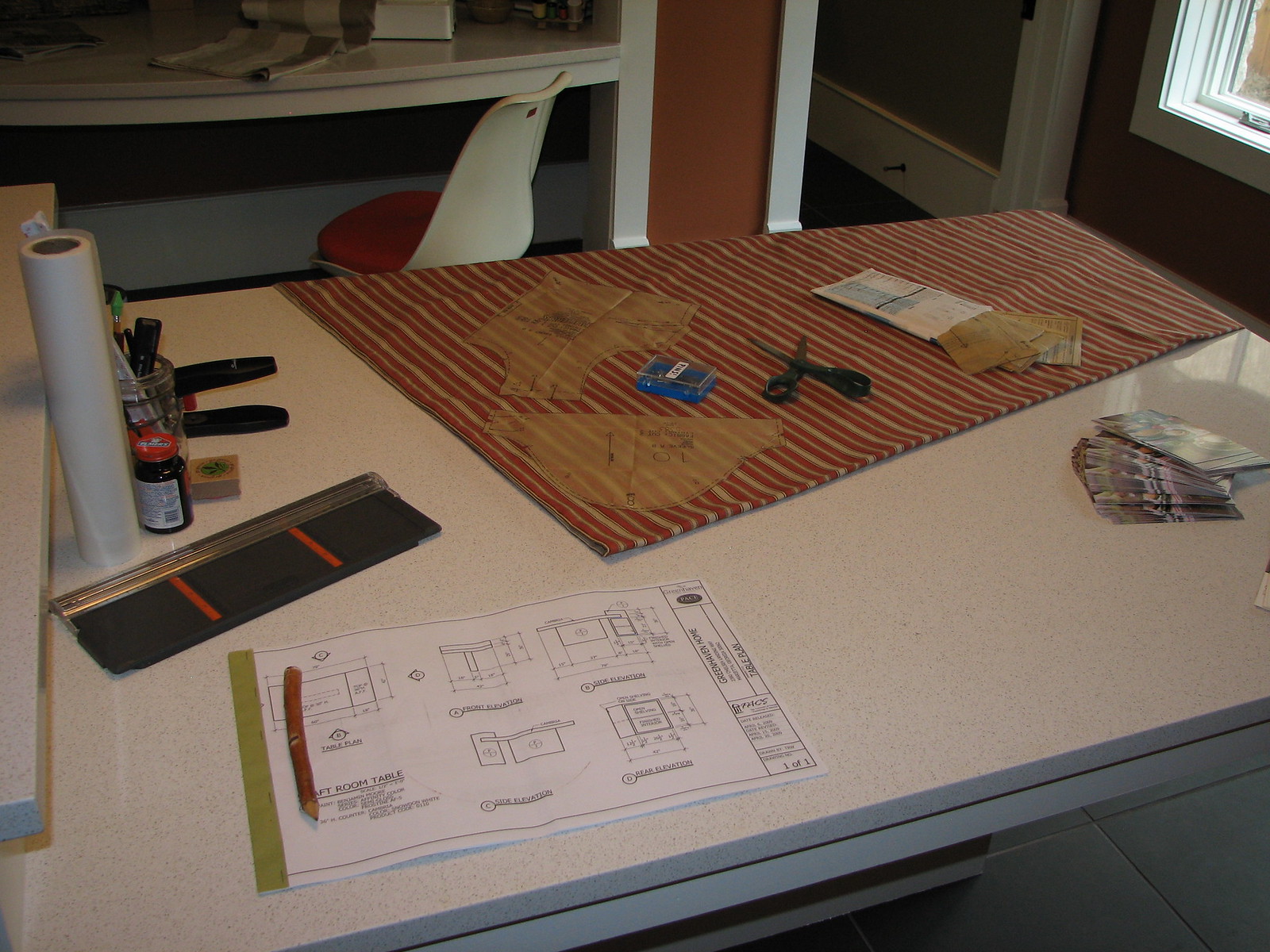This detailed photograph captures a well-organized work desk set up for a sewing project. The desk, made of white material with brown speckles, possibly quartz or granite, has an array of tools and materials neatly arranged on it. In the foreground, dark red fabric with light tan stripes is spread out, topped with pattern pieces ready for cutting. Nearby, there is a pair of scissors, a box of pins, and the pattern's packaging envelope. 

Additionally, the desk holds a cluttered pile of indistinguishable flyers, an architectural drawing overlaid with a thick brown pencil, and a standing roll of paper. A bottle of rubber cement sits next to a clear jar brimming with pencils, pens, and a ruler. Another notable object is a black, rectangular measuring device, approximately 12 inches by 4 inches. 

In the background, a second desk supports a white plastic chair with an orange seat. This desk holds more white fabric and what appears to be the base of a white sewing machine. The room features reddish-orange walls with contrasting white trim around doors and windows, enhancing the creative atmosphere of this sewing workspace.